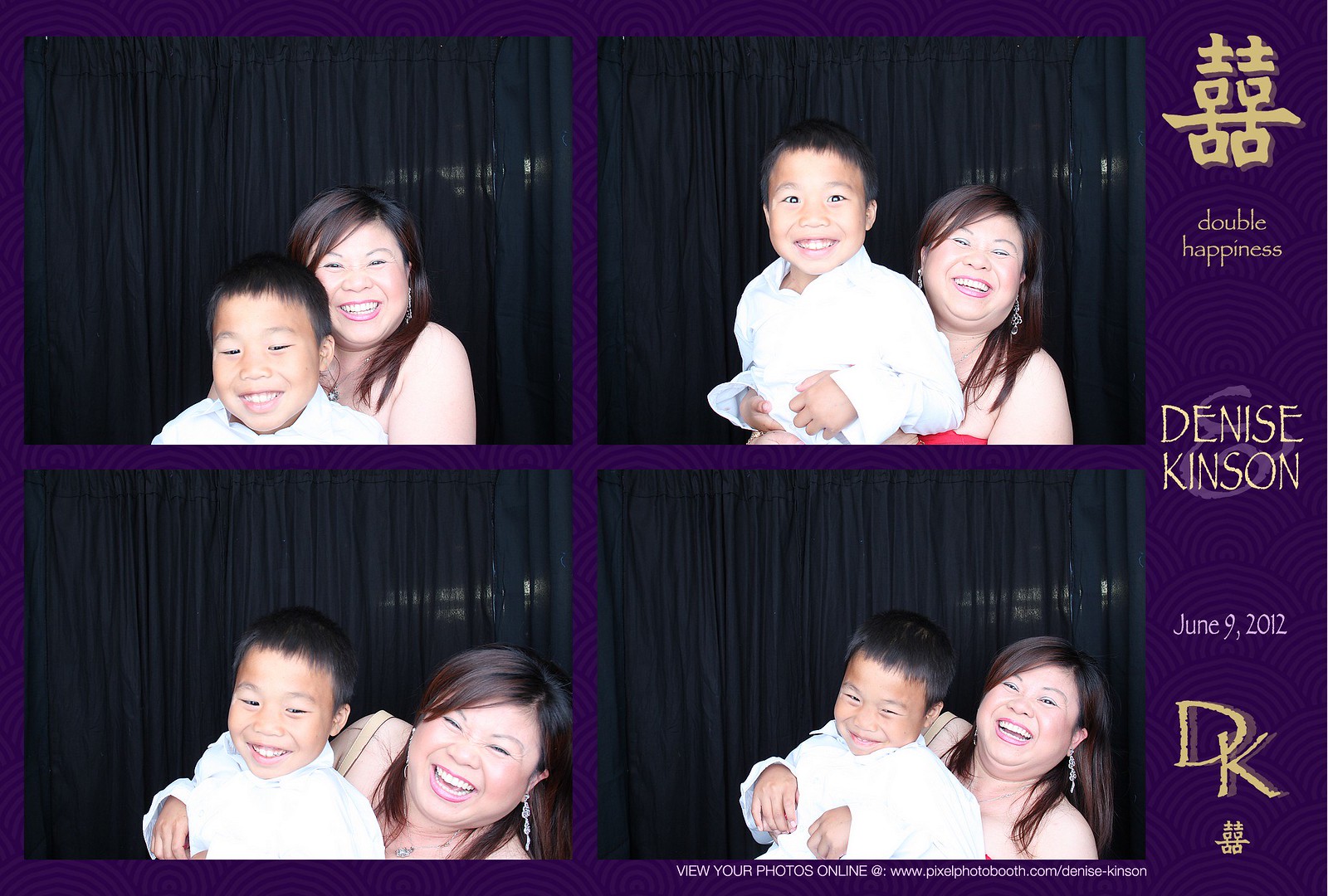This image features a grid of four well-lit photo booth photographs, capturing playful and joyful moments between an Asian woman with brown hair and an approximately 10-year-old boy with black hair. They are both smiling and appear to be having a great time, perhaps at a fair. The woman is dressed up, accessorized with earrings, and comfortably dressed for warm weather. Each photograph has a consistent black curtain backdrop. The purple border surrounding the photos includes text that reads "Double Happiness," "Denise Kinson," "June 9, 2012," and it instructs viewers to view their photos online at "www.pixelfotobooth.com/DeniseKinson."